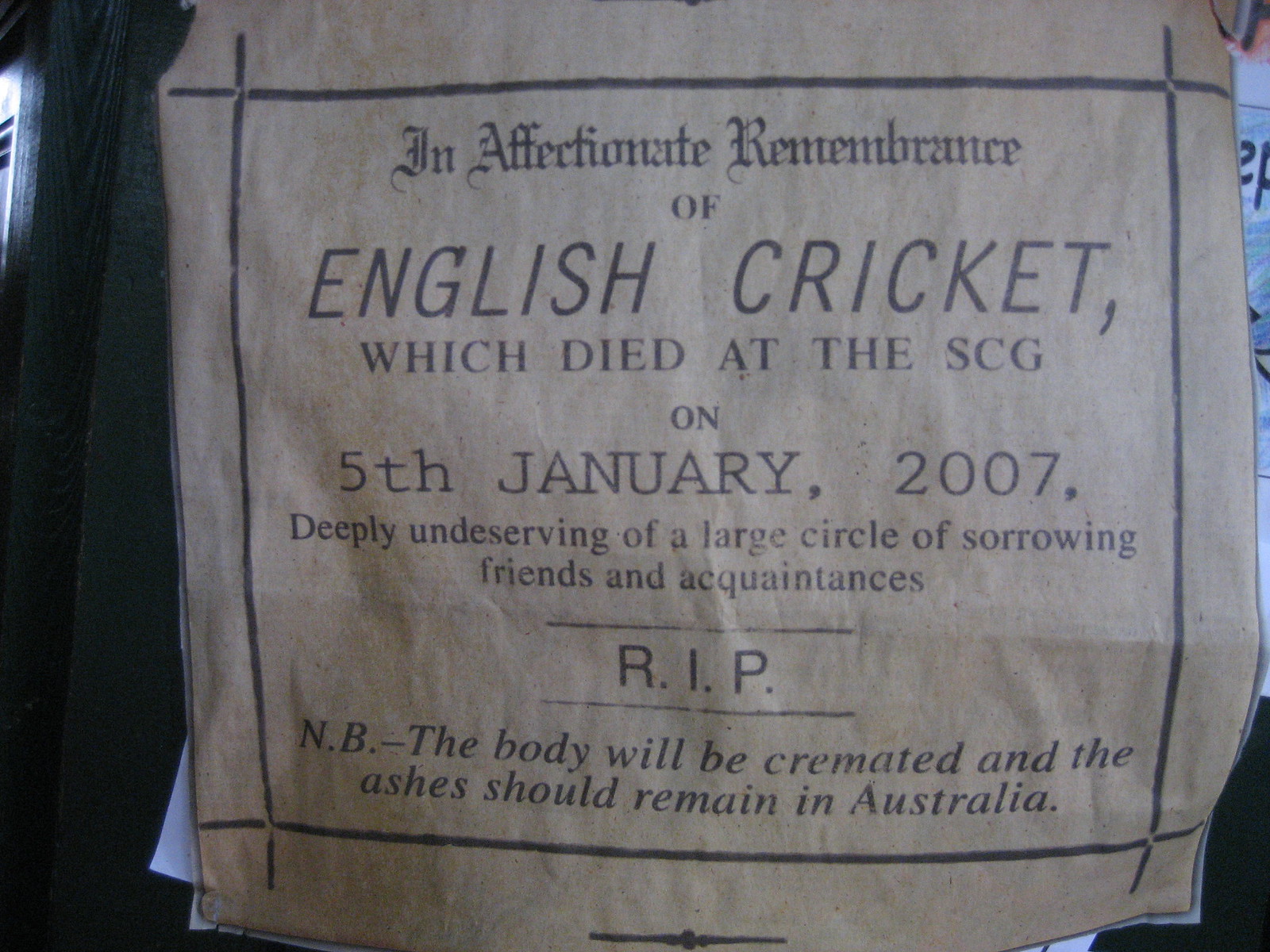The image depicts a cloth-like sign with a white background and black writing, dedicated as a memorial piece. The sign reads, "In affectionate remembrance of English cricket, which died at the SCG on 5th January 2007, deeply mourned by a large circle of sorrowing friends and acquaintances. Rest in peace. NB: The body will be cremated and the ashes shall remain in Australia." The sign has a border around it, and the entire photo is dominated by this sign. The background behind the sign appears to be a dark gray, possibly resembling a plaque, adding a somber tone to the image.